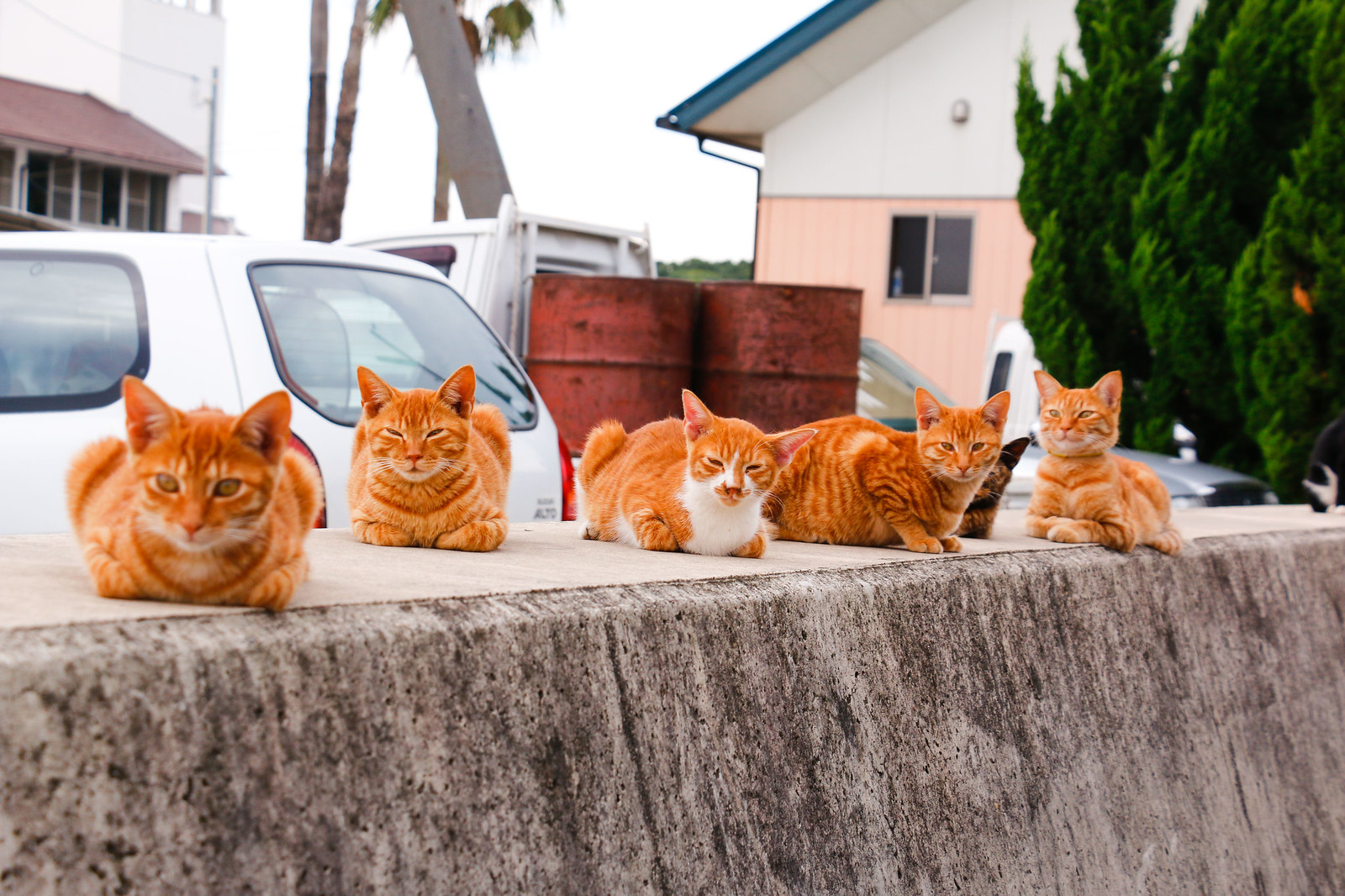This outdoor photograph captures six cats lounging on a grey stone wall, basking in the sunlight. Predominantly orange and white, five of the cats are clearly visible, their bodies aligned almost in a straight line and all intently gazing towards the viewer. The sixth cat, darker and tabby-colored, is somewhat hidden between the fourth and fifth cats from the left. The one central cat features a largely white underbelly, distinguishing itself from its orange companions. 

In the background, a bustling scene unfolds. A white delivery truck, bearing two rusted steel drums, is parked beside a white hatchback car on the far left. Partially obscured behind these vehicles, a silver car peeks through. Amidst these elements, vibrant greenery frames the right side of the image, with several tall, leafy trees adding a touch of nature. The backdrop features a two-story house painted in shades of pink and white with a blue roof trim, along with a building on the far left that has a light reddish-brown roof and black window shutters. The sky overhead appears bright and white, emphasizing the vivid colors below.